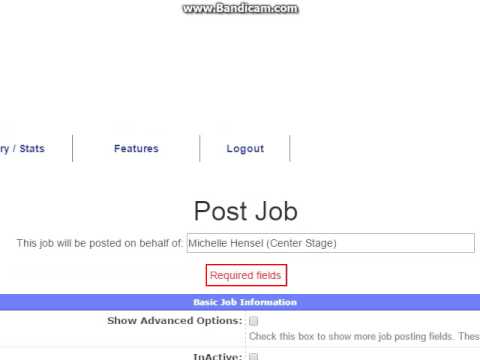In the image, a screenshot is displayed against a white background. At the top center of the screenshot, "www.bandacam.com" is written in block text. Beneath this, in blue text, it reads "ry/stats" (with "ry" denoted as "R" forward slash "Y"), followed by a dividing line, "features," another dividing line, and then "logout." Below these sections, centrally located in larger black text, the phrase "Post Job" is prominently shown. It also mentions that the job will be posted on behalf of Michelle Hensel. Centrally positioned on the screen, a red-bordered box with red text states "Required Fields," and just below it, "Basic Job Information" is visible. Additionally, white text on a blue background indicates "Show Advanced Options," with a checkbox next to it for displaying more job posting fields, which is marked as inactive.